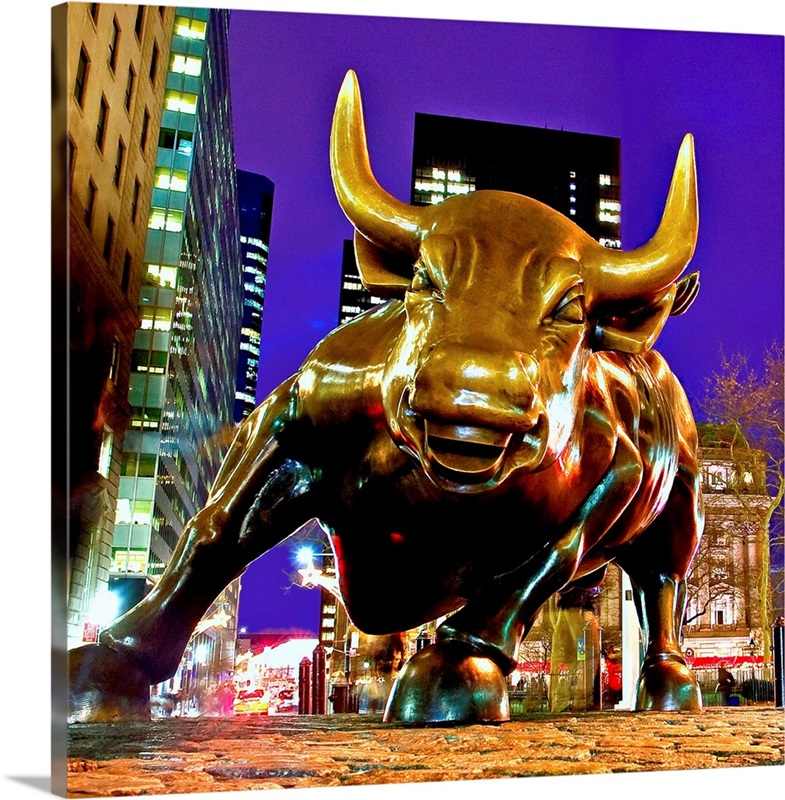This image captures the iconic bronze bull statue near Wall Street, known as the Bowling Green Bull. The photo, approximately five inches square, displays the bull in exquisite detail from a lower perspective, as if it's charging towards the camera, creating a sense of dynamic motion. The bull, leaning slightly to the right with its front legs tilted, seems almost to be smiling, its polished, gold-tinted horns and nose gleaming in the night, a testament to the countless tourists who have touched them. It stands on a brick pavement amidst a bustling New York street. Behind the bull, tall skyscrapers with illuminated office windows and some shorter buildings and shops are visible, bathed in the soft glow of multi-colored lights reflecting off the metallic surface of the statue. Above, the sky is a deep, dark purple, adding to the vibrant and lively atmosphere of the scene.